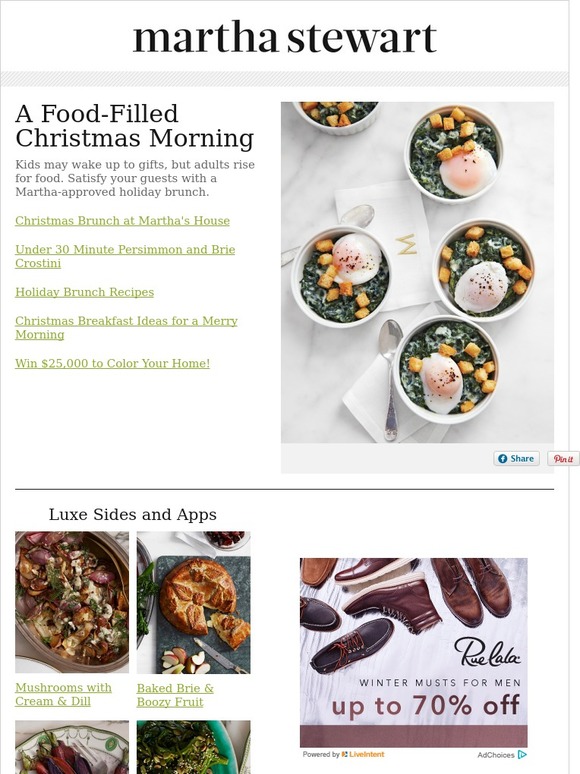The top of the image prominently features "Martha Stewart" written in black. It vividly captures the essence of a food-filled Christmas morning, emphasizing that while children may eagerly wake up to gifts, adults look forward to delicious food. The caption invites you to satisfy your guests with a Martha Stewart-approved holiday brunch, boasting dishes like persimmon and briar crostini. Highlighting the ease of preparation, it promises a festive Christmas brunch at Martha's house in under 30 minutes.

The image also teases holiday brunch recipes and Christmas breakfast ideas designed to make your morning merry. In one corner, there's a mention of a contest to win $25,000 to refresh your home's color scheme. Various food and dessert items are showcased, hinting at delectable dining options. On the bottom right, there's an advertisement for winter shoes for men, offering up to 70% off, courtesy of Life Intents. The image palette features a harmonious blend of green, white, black, and brown.